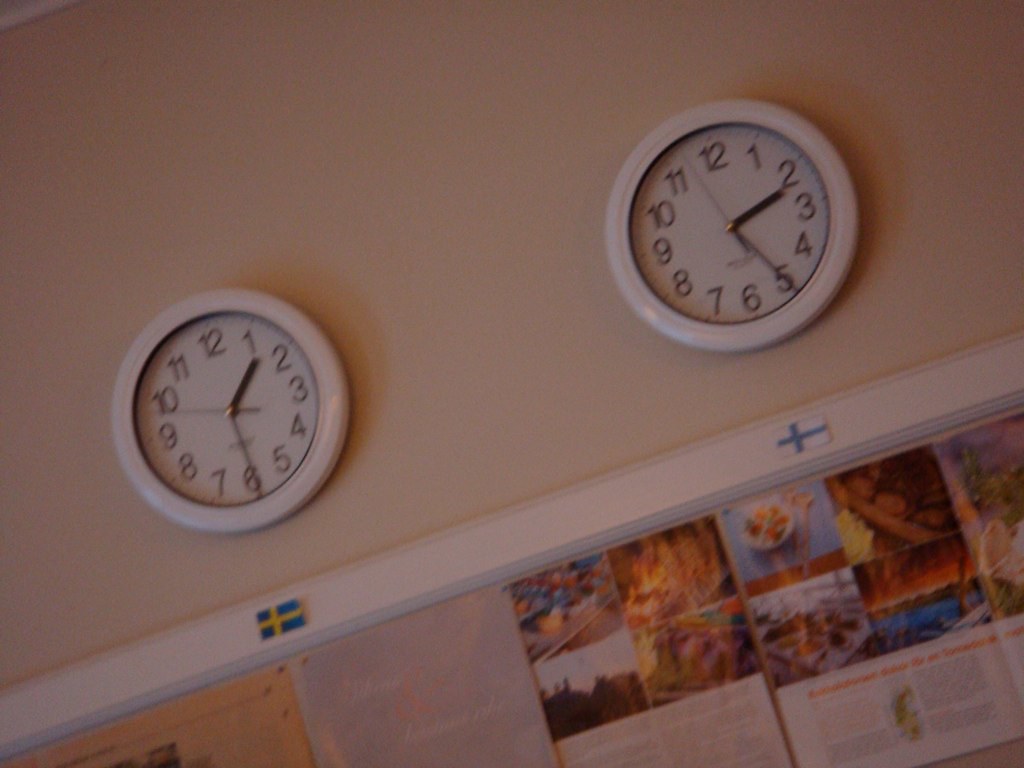The photograph depicts a slightly diagonal view of an off-white wall adorned with two identical white clocks. Both clocks feature black numerical markings and hands, including the seconds hand. The clock on the left shows a time of 1:30, while the one on the right indicates 2:25. Below them are two flags: one under the left clock is a blue background with a yellow cross, and the other under the right clock is a white rectangle with a blue cross. These flags are accompanied by a bulletin board with a white wooden frame, displaying numerous pages from magazines or newspapers. The pages contain colorful images, including a picture of a fire and a bowl of vibrant food, along with dense text. Shadows cast partially over the wall and the bulletin board, adding a touch of depth to the scene.